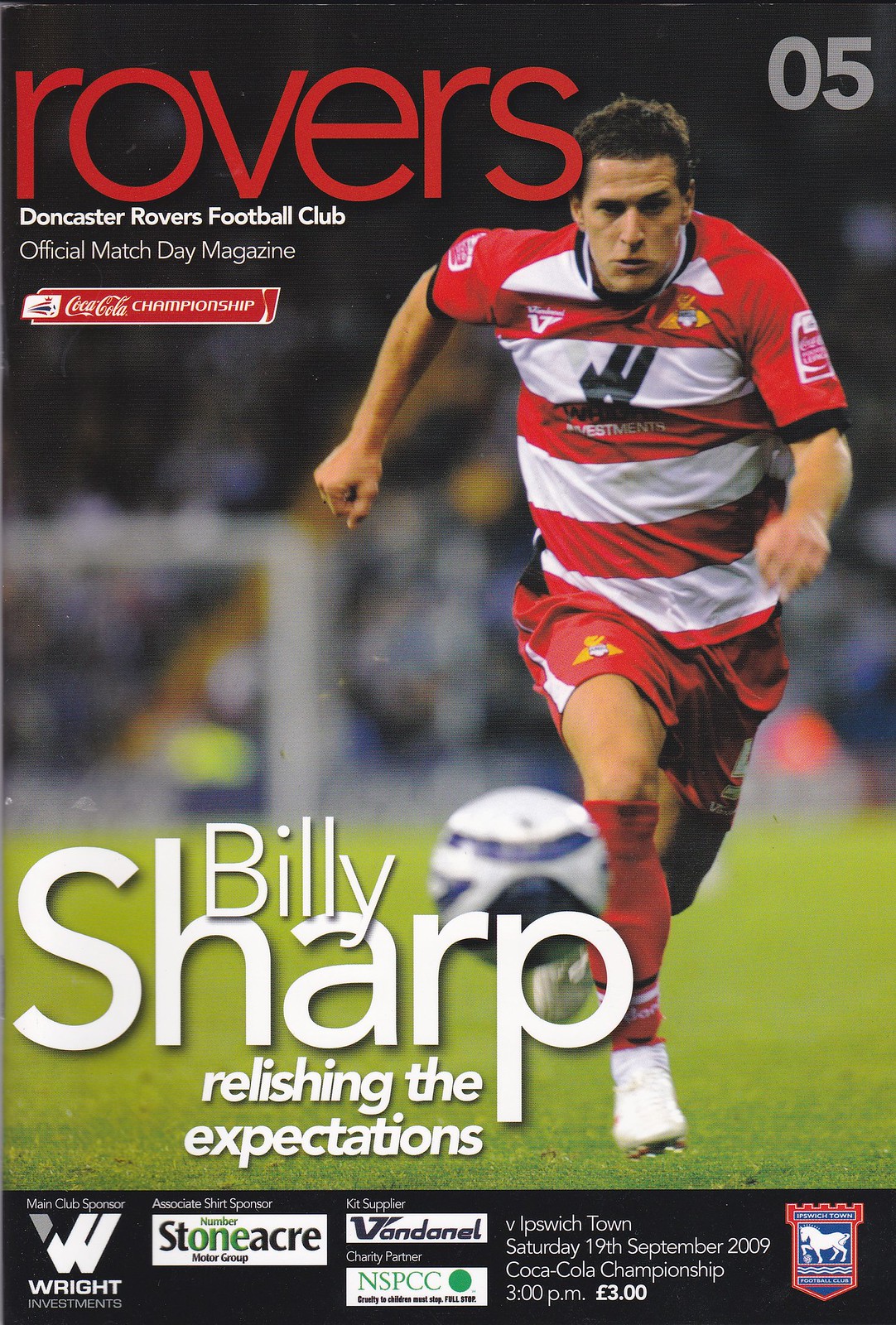The image is the front cover of a football program magazine, prominently featuring a male soccer player running towards the camera while chasing a ball on a green pitch. He is dressed in a red and white striped jersey, red shorts, long red socks, and white cleats. In the background, the soccer goal and grandstands, likely filled with spectators, are blurred out. At the top of the cover, set against a darkened backdrop, "Rovers" is written in bold red text. Just below, in white text, it reads "Doncaster Rovers Football Club Official Match Day Magazine." The upper right corner features a "05." Further down, the cover showcases the Coca-Cola Championship logo. Dominating the central portion, it has "Billy Sharp, relishing the expectations" in large white text. At the bottom, a black bar contains various sponsor logos, including Stoneacre and Wright, along with additional details: "V. Ipswich Town, Saturday, 19th, September 2009, Coca-Cola Championship, 3 p.m., 3 pounds."